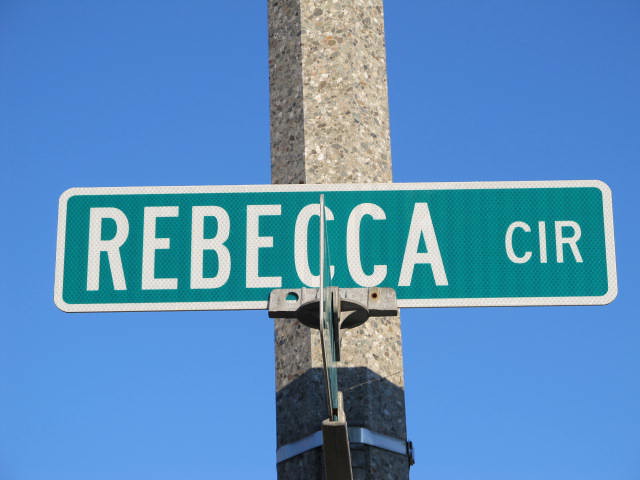This zoomed-in photograph captures a metal pole at the center, extending beyond the frame both at the top and bottom, making it impossible to determine its full height. The pole is predominantly grey, peppered with white and brown specks, and features a shadow at its base. Affixed to the pole with metallic straps is a rectangular, horizontally oriented street sign that is green with a white border and text, displaying "REBECCA CIR" in all capital letters. The green sign contrasts sharply with the bright blue, cloudless sky in the background. Below this sign, another road sign is mounted vertically facing right, though its details are not legible.